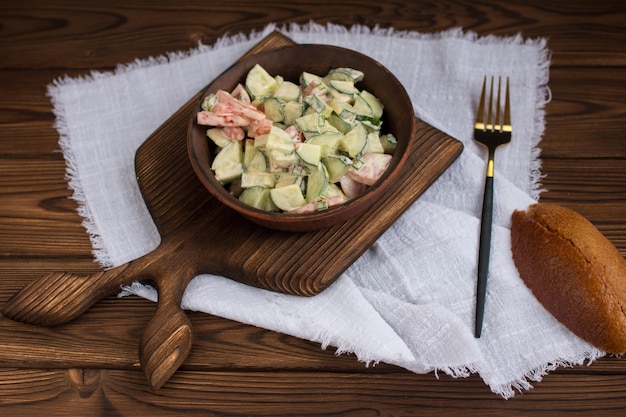The image captures a rustic and artistically arranged food setting. At the center, a brown wooden planked table serves as the backdrop, partially covered by a folded, uneven-edged white linen napkin. Placed diagonally atop the napkin is a wooden cutting board featuring a unique dual-handle design resembling a fish tail. Resting on this board is a small wooden bowl filled with a colorful mixture of diced cucumbers, tomatoes, and possibly onions, all dressed in a creamy sauce. To the right of the bowl, a gold fork with a wooden handle is neatly positioned. In the lower right corner of the image, a deep brown, rounded loaf of bread with a slight crack in its crust adds a touch of rustic charm. The predominant colors are the natural browns of the wooden elements and bread, the white of the napkin, and the vivid greens and reds of the salad, creating a visually appealing and inviting scene.